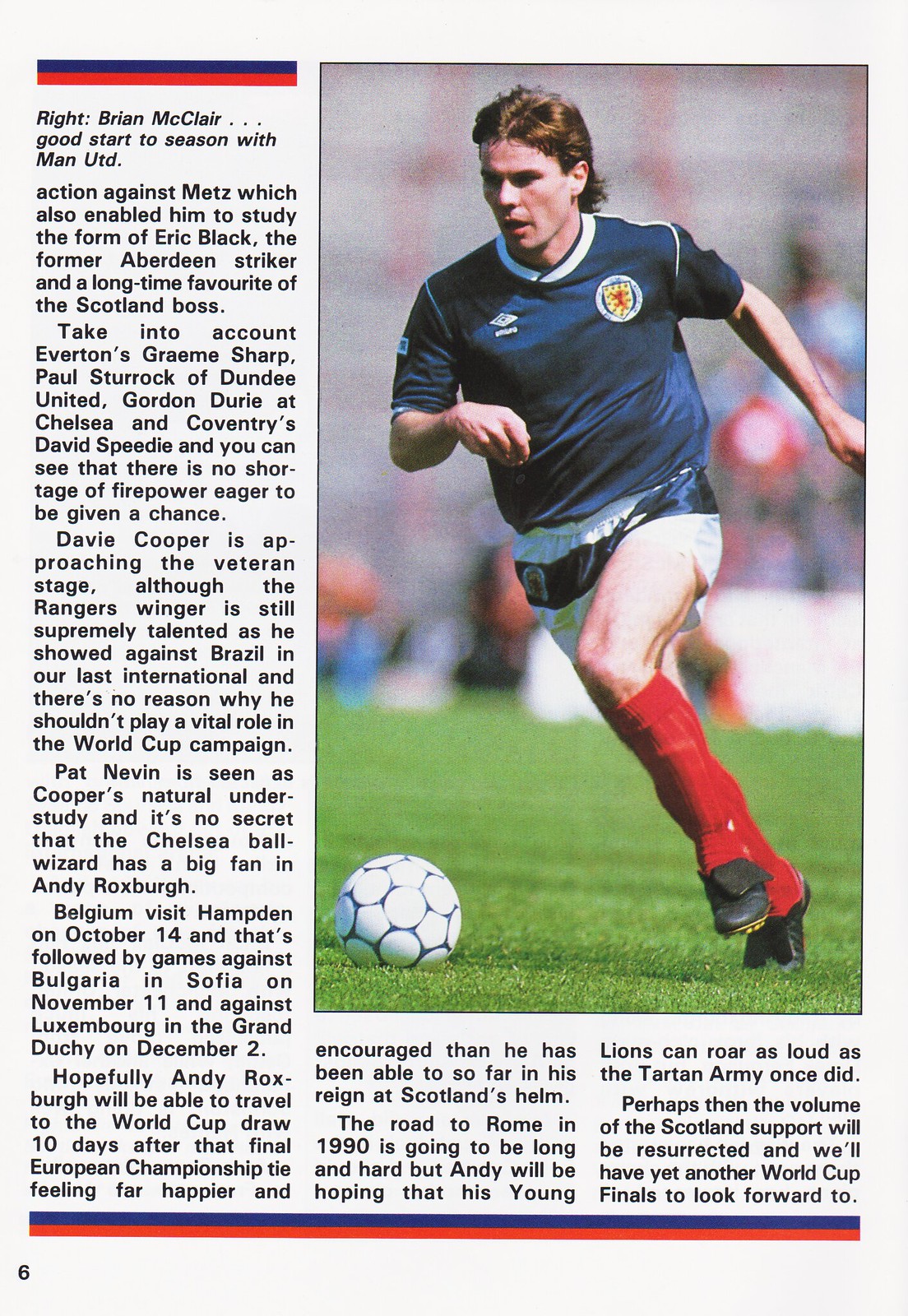The image accompanying the article depicts a clean, scanned page from a soccer magazine, marked as page six in the lower left-hand corner. The page is bordered by distinctive blue and red stripes, with the border continuing partially along the first column but not the other two. The article itself lacks a title and features a photograph that dominates the two right-hand columns, underneath which lie two small paragraphs of text. 

The prominently featured color photo captures a young male soccer player with short, reddish-brown hair, dressed in a dark blue, short-sleeved jersey with a white collar and a circular emblem on the left side of his chest showcasing a red and orange lion. He is also wearing white shorts, red socks, and black and red cleats, running on a grassy field. The action shot shows him poised to tackle or kick a soccer ball with blue and white patterns. 

The textual content of the article begins on the left side of the page and starts with, "Brian McClare: Good start to his season with Man Utd." It continues by describing his actions against Mets, which provided an opportunity to study the form of Eric Black, a former Aberdeen striker and a celebrated figure in Scotland. The print is in black on a white background, with the text from the first column continuing to the right underneath the large photograph.